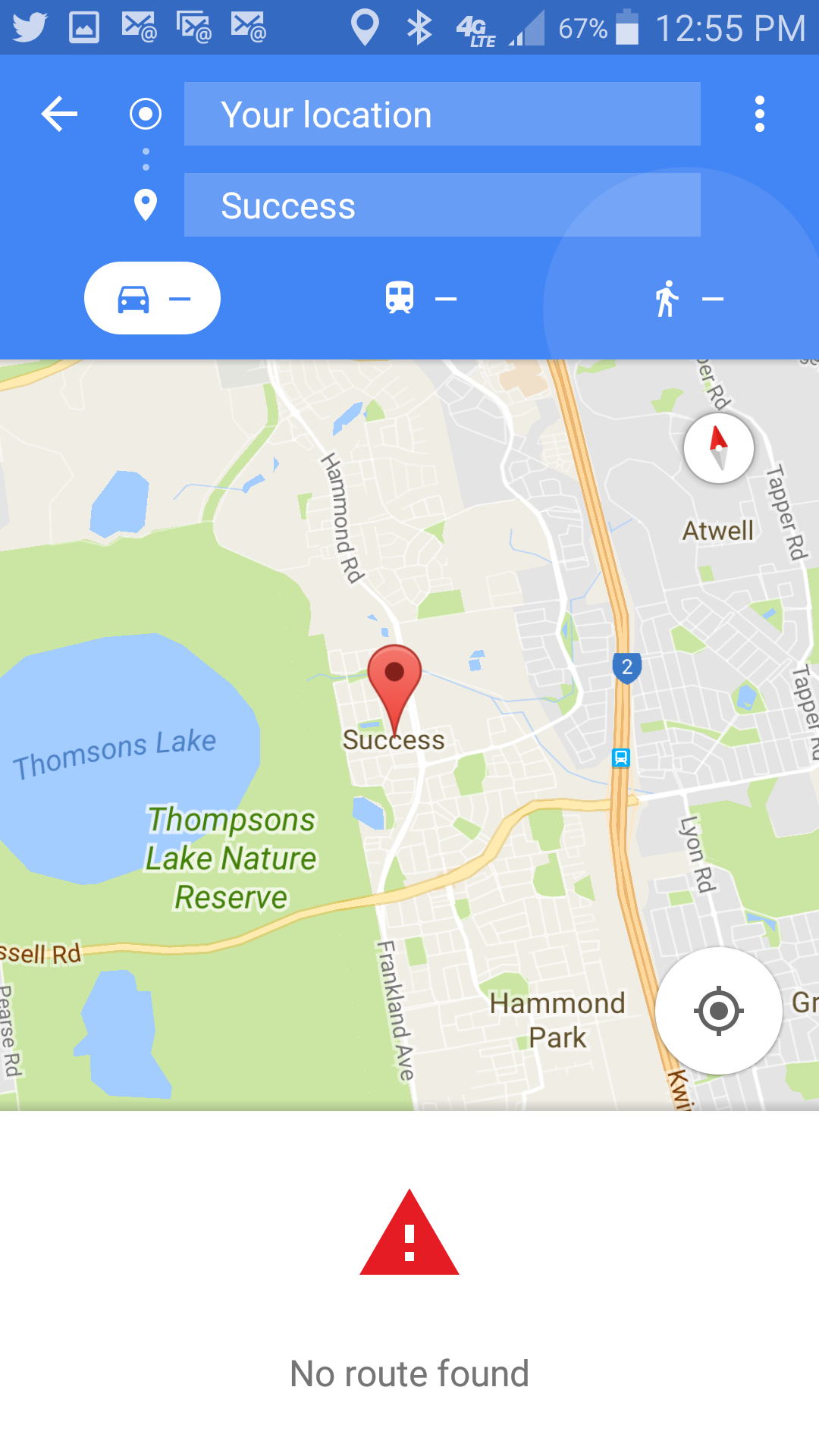This image is a Google Maps screenshot, capturing a detailed overview of a specific location. 

At the top of the screenshot, a dark blue bar displays several icons indicating various functionalities and statuses. From left to right, the bar includes an old Twitter white bird icon, a square box with a mountain range symbol, three envelopes with "@" symbols over them, a location icon, a Bluetooth symbol, a 4G LTE indicator with two bars of signal strength, a battery icon showing 67% battery level, and the current time displayed as 12:55 PM.

Below this bar, a blue box contains navigation options with a white arrow, a white circle, and a white location pin icon. This box reads "Your location," followed by the word "Success" in a white text. Adjacent to these, two smaller boxes display icons for car, bus, and pedestrian directions. To the right of these boxes, three vertical white dots suggest additional menu options.

The map itself occupies the main portion of the image with a diverse color scheme, featuring shades of tan, green, blue, and gold. Prominent features within the map include a red arrow, various street delimitations, white and gold street lines, and a body of water labeled "Thompson's Lake" in blue text. Green text indicates "Thompson's Lake Nature Preserve." Key roads and landmarks are present in gold, while a red pin labeled "Success" marks a specific location nearby "Hammond Park" and "Lion Road."

At the bottom of the map, a white circle with a gray bullseye symbol sits alongside a red triangle containing a white exclamation point; this section reads "No route found" in gray text, indicating navigation issues.

This descriptive caption precisely details all visible elements in the Google Maps screenshot, providing a comprehensive understanding of the image's content.